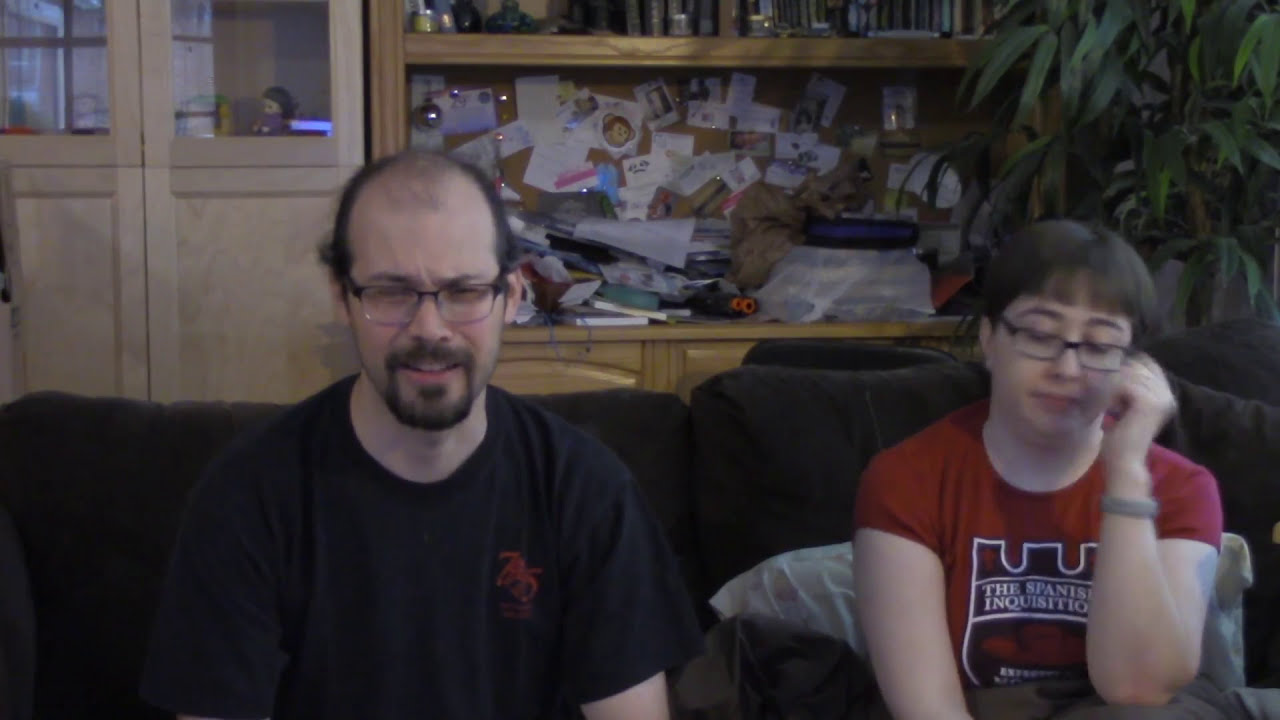In the image, two individuals are seated on a dark-colored, possibly black or dark brown, couch. Both individuals are Caucasian and are positioned about one foot apart from each other. The man on the left has a mostly bald head with some hair on the sides and back. He sports black, square-framed glasses and a goatee. He is wearing a black t-shirt and appears slightly slouched, with his mouth partially open, displaying a confused expression as if uncertain about what he is watching on TV. To his left, on the right side of the image, is a teenage boy with medium brown hair, also wearing black glasses. He is dressed in a tight red t-shirt and has a slightly chunky build. The setting includes a cluttered, wooden built-in shelf filled with a miscellany of items visible in the background. The couch also appears to have some pillows or sheets placed in the middle area between them. On the left side of the image, a pale wooden china cabinet is present, and on the right side, there are glimpses of plant leaves.